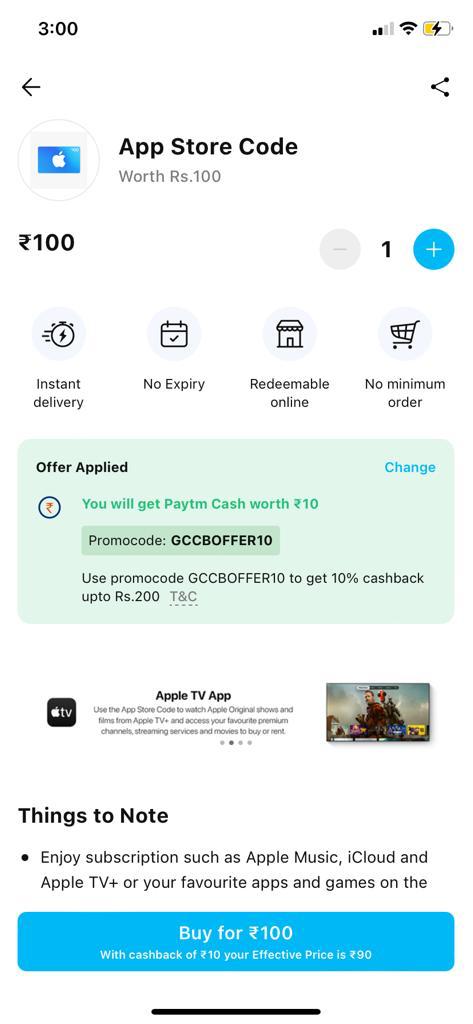This is a screenshot from a mobile phone displaying a shopping interface. The background is predominantly white. In the top left corner, the black text indicates the time as 3:00. The top right corner features several status icons: a charging battery outlined with the left side yellow and the right side white, a full Wi-Fi signal, and a full Internet 2.0 signal. To the right of these icons is a black share icon, and to the left, there's a black arrow pointing to the left. Below these icons, a white circle with a thin gray border contains a blue square with a white apple inside.

To the right of this emblem, bold black text reads “APP Store Code.” Directly below, smaller black text states “Worth RS.100.” On the left, bold text shows “100,” while the right side features a blue circle with a white plus sign. Next to it is a black number “1” followed by a gray circle with a darker gray minus sign. Further down, there are four clickable icons with labels below them. From left to right, these read: “Instant Delivery,” “No Expiry,” “Redeemable Online,” and “No Minimum Order.”

A blue tab in the bottom left corner says “Offered Applied” in dark, bold text, while to the right, blue text reads “Change.” Further left, a black circle with an unclear red symbol inside is too small to discern clearly. To its right, green text says “You will get cash P-T-P-A-Y-T-M cash worth $10.” Below, there is a promo code followed by instructions to use the promo code to get $10 cash back.

Further down, the Apple TV logo appears on the left, followed by information about Apple TV and an image of a show. Beneath this, black-bordered text says “Things to Note,” with two lines of additional information. At the bottom, a blue tab stretches across the screen, stating "Buy for $100" in white text. Below this, another line in white notes, "With cashback of $10, your effective price is $90."